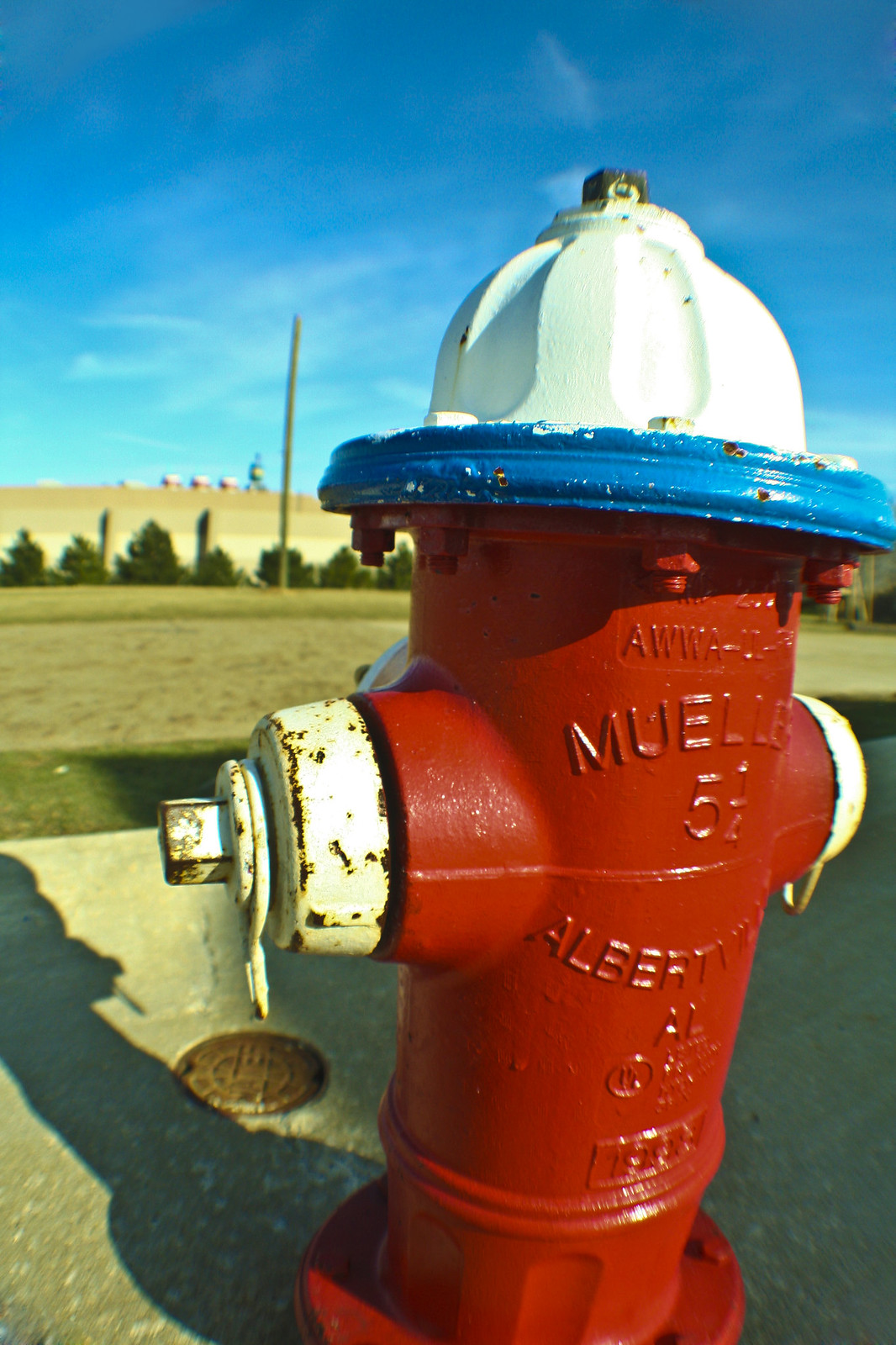This vibrant image showcases a red fire hydrant with distinct white spouts and a blue ring topped with white. The hydrant stands on a cement platform and casts a shadow to its left. The setting appears to be a desolate, perhaps desert-like area, featuring a barren field with sparse, dry grass and some green shrubs. The backdrop includes a vividly blue sky with light cloud coverage and the tops of distant, multi-colored buildings that are red, white, blue, and yellow. A three-colored wall in medium brown, light tan, and white, along with green hedges, forms part of the background. There is also a rusted, small manhole in front of the hydrant. Additional elements include a line post with electrical wires and possibly barns or small buildings along with a water tower faintly visible in the distance. The fire hydrant bears intricate inscriptions including "A-W-W-A Mueller" and the partially visible word "Albert."